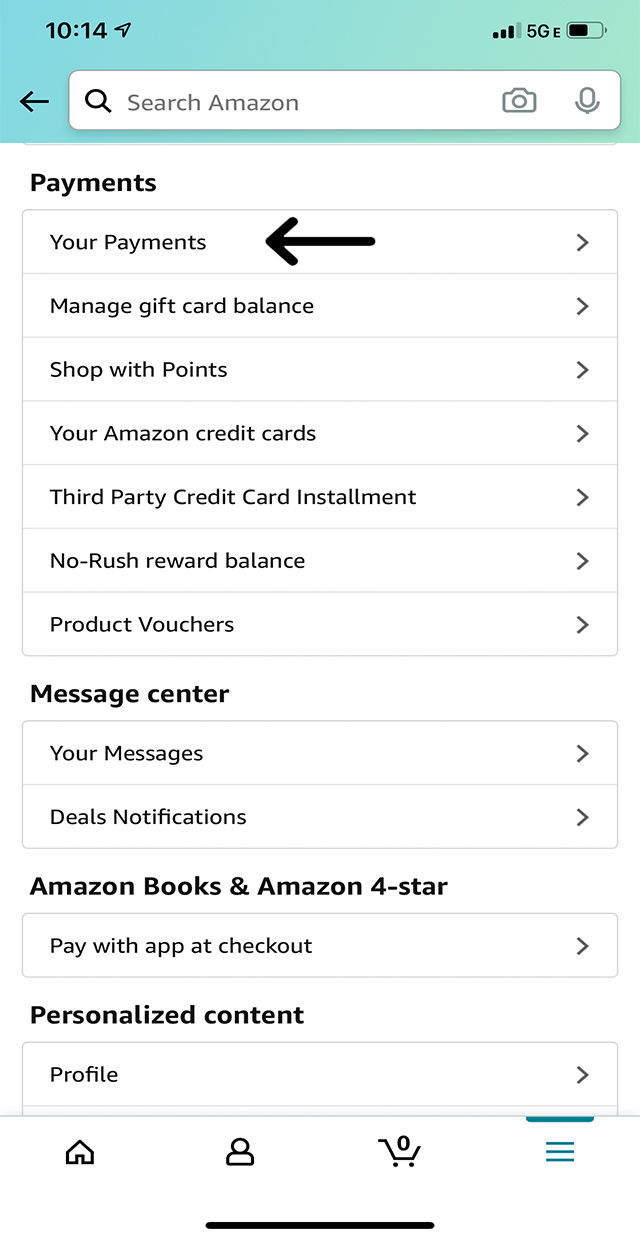This image is a detailed screen capture of the Amazon mobile app, taken from a smartphone. In the upper right-hand corner, visible indicators include Wi-Fi signal bars, a 5G network symbol, and a battery icon. The top of the screen features a minty turquoise-green bar beneath which lies the text box labeled "Search Amazon." 

Central to the screenshot is a section likely part of a how-to guide, emphasizing the "Your Payments" subheader under the primary header "Payments." This subheader is highlighted by a black arrow pointing left, drawing attention to it specifically. The display also includes other main headers such as "Message Center," "Amazon Books," "Amazon Four Star," and "Personalized Content."

At the bottom of the screen, the navigation bar showcases several icons: a home icon, a user profile icon, a shopping cart icon, and a hamburger menu icon. Notably, the screen is void of any images, focusing solely on various navigational and informational elements of the Amazon app pertinent to user account management.

This screenshot is best described as part of a tutorial, presumably illustrating the process for accessing payment information on the Amazon app.